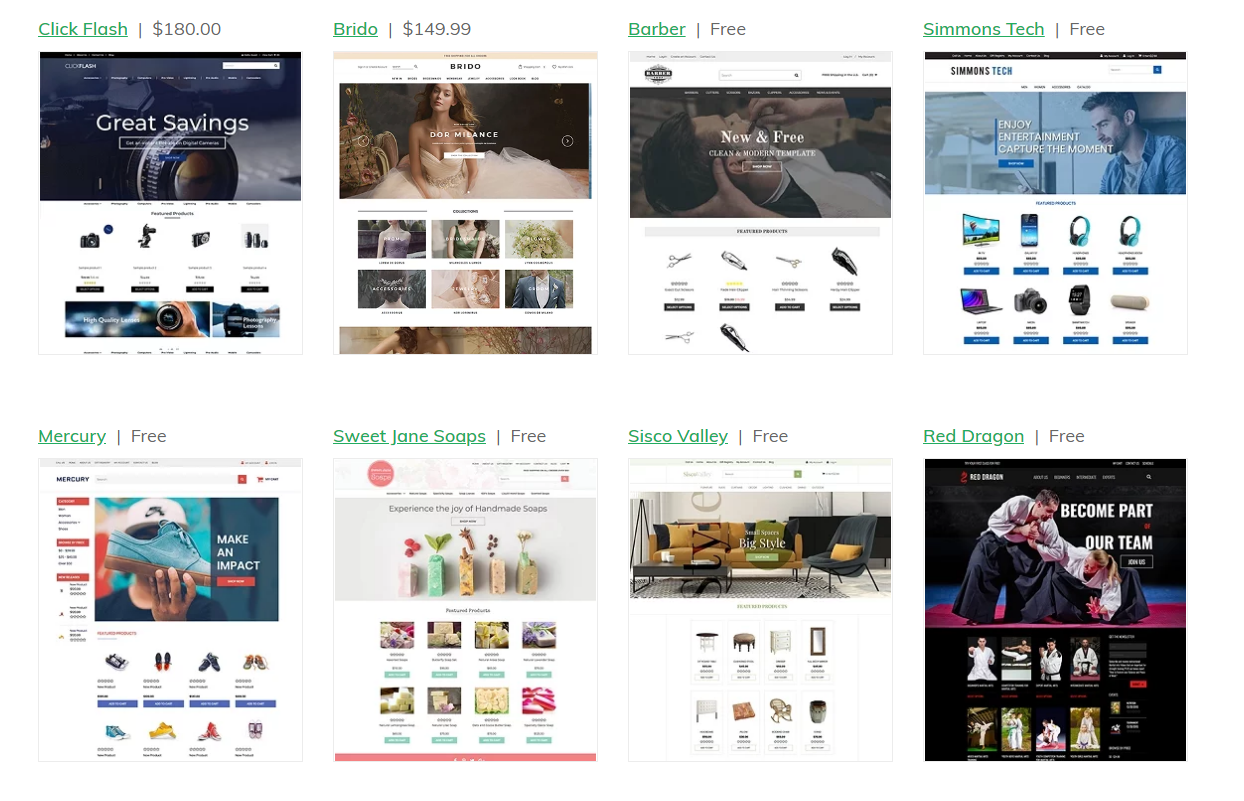This image features a composite of eight small webpage screenshots arranged in a grid layout on a white background. Each individual screenshot represents sections of different webpages, devoid of any headers, footers, or borders. The presentation is two rows of four screenshots each. Text elements within these images are underlined and displayed in green.

The top row consists of:

1. **Click Flash** - Priced at $180. The screenshot includes a horizontal photograph at the top, followed by additional product or styled photographs.
2. **Brido** - Priced at $149.99. Similar structure with a top horizontal image and subsequent product visuals.
3. **Barber** - Offered for free. It retains the same layout of a top photograph with following visual aids.
4. **Simmons Tech** - Also free, featuring the same layout design as the others.

The bottom row consists of:

1. **Mercury** - Free of charge. Includes a horizontal image at the top with further photographic details below.
2. **Sweet Jean Soaps** - Free. Maintains the same webpage structure.
3. **Cisco Valley** - Free. Displays the typical layout with a top photograph and supporting images underneath.
4. **Red Dragon** - Free. However, this specific screenshot deviates by having a black background, unlike the white backgrounds of the others. The visual content layout remains consistent with the group.

Each of these screenshots appears to represent website advertising content, showcasing various products and styled images. The composite nature of this image highlights different online storefronts or promotional material in a cohesive manner.